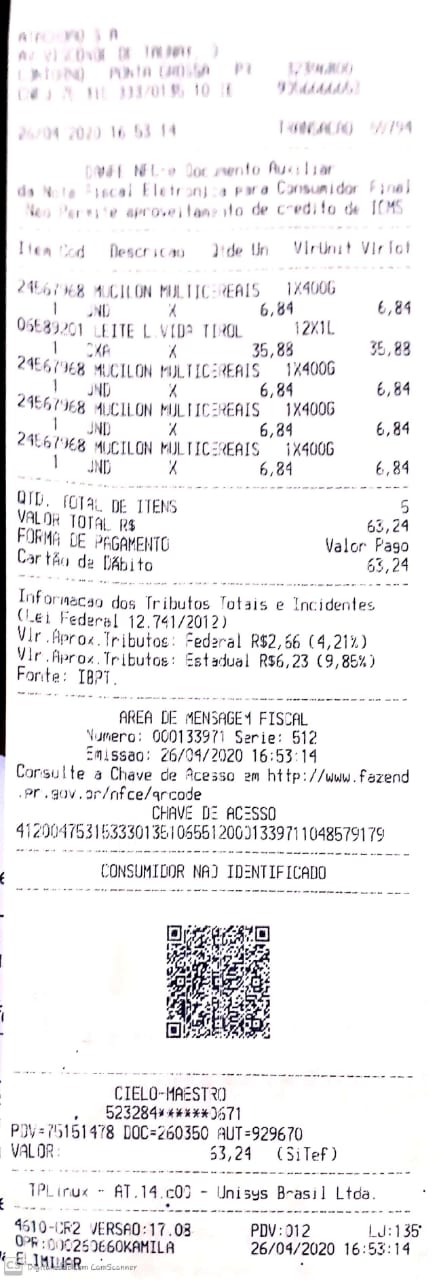This vertically-oriented photograph displays a somewhat blurry receipt from a non-U.S. country, potentially Brazil, based on the appearance of the word "BRASIL." The receipt contains numerous items listed in Spanish, although the text is difficult to read. The left-hand side of the receipt features a black border running down the top two-thirds beside the item listings. Key details include a sequence of monetary amounts: $6.84, $35.88, and multiple instances of $6.84, leading to a total purchase amount of 68.24. There is also a QR code positioned towards the lower center of the white receipt with black print. Noteworthy codes such as PDV-012 and LGA-135 are present, along with a reference to "Aria de Mensaje 1 Fiscal" and a website URL: www.fazendpr.gov.org. Additionally, the date on the receipt is marked as 26/04/2020.